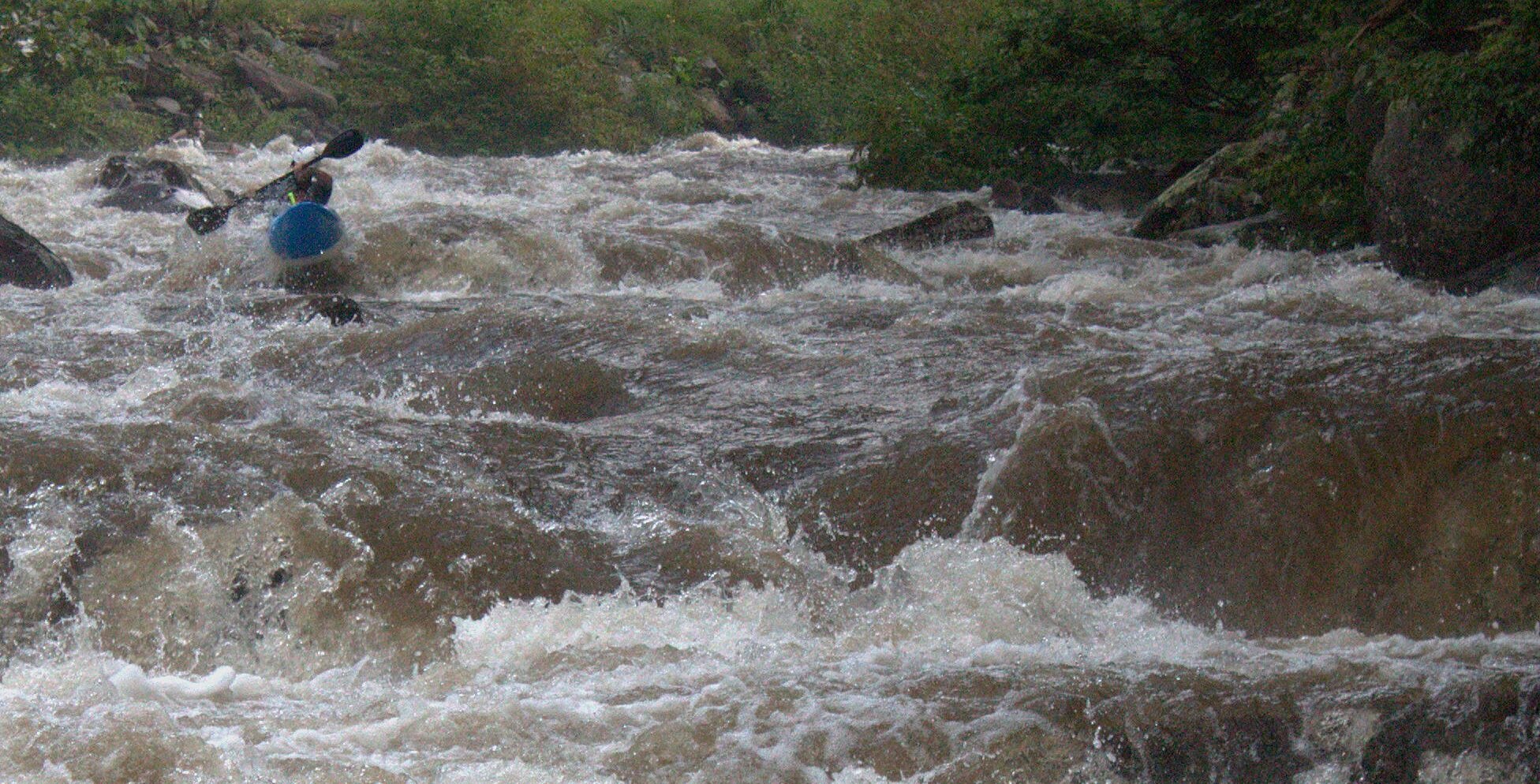The photograph captures an exhilarating scene of a kayaker navigating through a rushing river. The water is tumultuous and white-capped, indicative of the multiple levels and intense energy of the rapids. The kayaker, clad in a blue kayak, holds their paddle aloft as they maneuver through the choppy, dark brown waters. Surrounding the river are large boulders and patches of lush greenery, while the background features a hilly terrain dotted with trees. The scene conveys a sense of adventure and the rugged beauty of nature in motion.